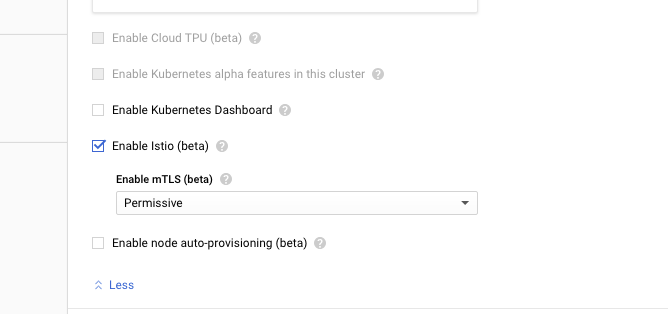This image displays a configuration settings page with several selectable options. The options available on this page include:
- "Enable cloud CPU" with an adjacent checkbox.
- "Enable Kubernetes alpha features in this cluster," offering advanced, experimental features with a checkbox.
- "Enable Kubernetes dashboard" with a checkbox to activate the GUI for managing and monitoring the cluster.
- "Enable Istio," indicated as a recommended setting for better service mesh management, with a checkbox.
- "Enable MTLS (Mutual TLS)," again noted as a recommended setting for enhanced security, with a selection for "Permissive" mode and a checkbox.
- "Enable node auto-provisioning," recommended for dynamic scaling of resources, with a checkbox.

There are no additional details or options presented on this configuration page.